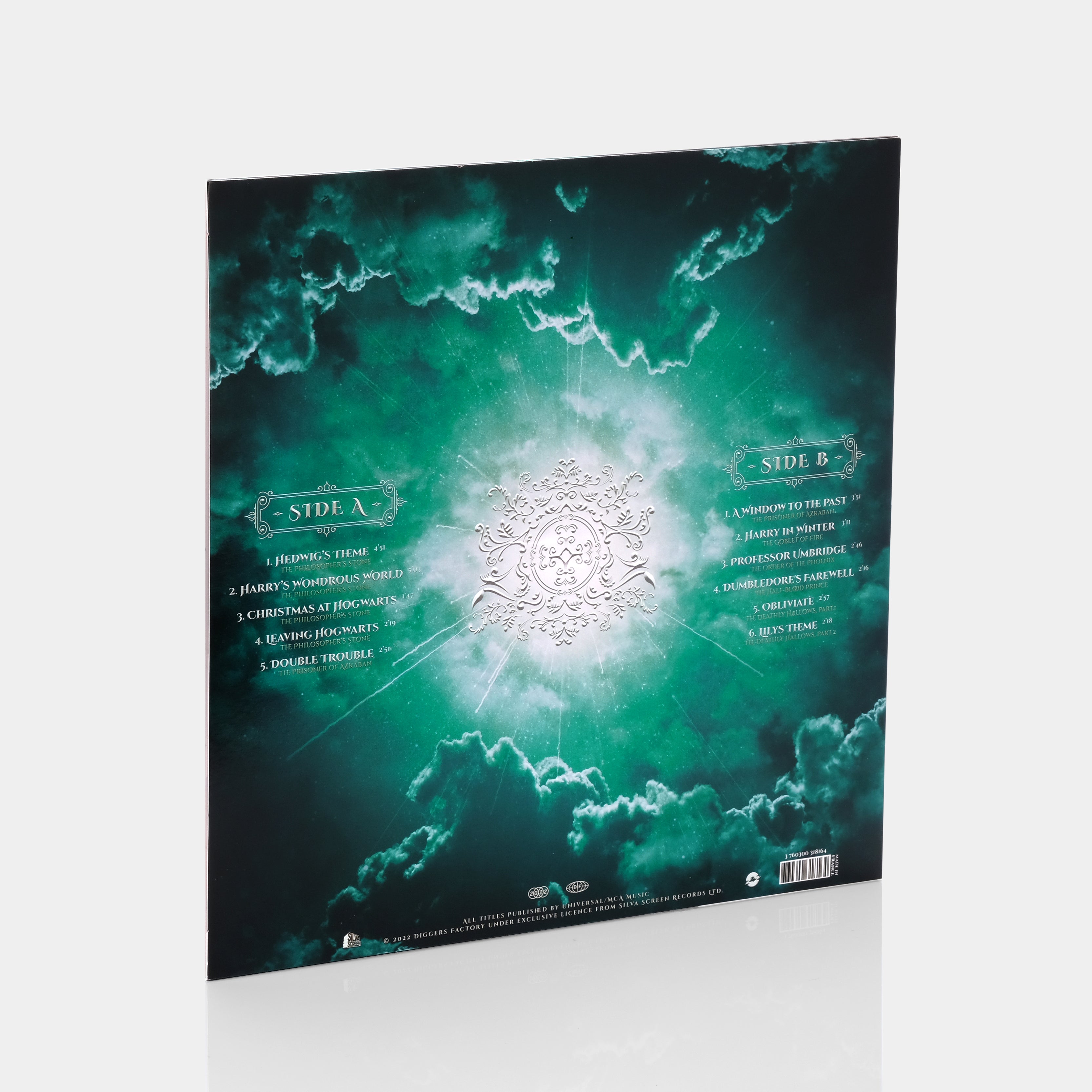The image showcases the back side of a Harry Potter soundtrack record, nestled against a light grey or purple background. The cover, which is a perfect square, possibly hints at a vinyl album. Dominated by hues of black and green that gradient into darker tones as they extend outward, the design centers on a mesmerizing scene of clouds in a mysterious, greenish-blue sky, evocative of a tumultuous, nighttime atmosphere. At the heart of this artwork resides a decorative metal emblem with scroll-like designs emanating from it, enveloped in an ethereal white aura. The track titles for Side A and Side B are listed on either side of this center image, though only a few can be discerned: number 3 on Side A is "Christmas at Hogwarts," and number 5 is "Double Trouble," while Side B includes "Harry's First Winter" as its second track. The record side lists indicate five songs on Side A and six on Side B. Fine white print adorns the bottom of the cover, featuring a small square with a scan code.